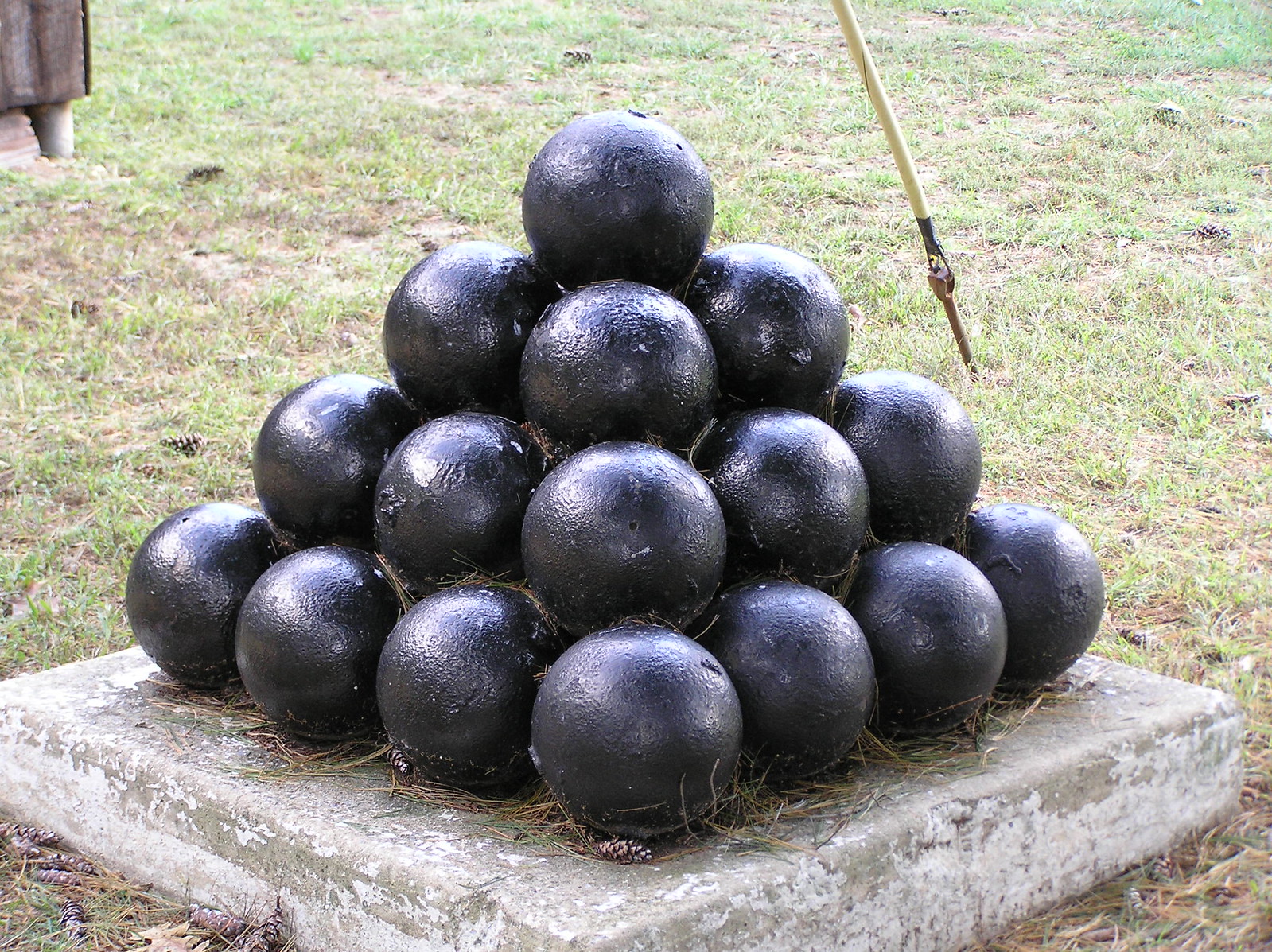This is a color photograph taken outdoors, depicting a decorative stack of black cannonballs neatly arranged into a pyramid shape. The base layer consists of sixteen cannonballs (4x4), followed by the next layer of nine cannonballs (3x3), with the subsequent layer featuring four cannonballs (2x2), culminating in a single cannonball at the top. The cannonballs rest on a light gray, stonewashed concrete pad that appears to be roughly five to six inches thick and shaped like a square. The setting is a grassy field with patchy areas, some of which are brown. Behind the stack, there is a yellow guide wire inserted into the ground, supporting a post or pole. In the background, an outdoor furniture piece with brown legs and a brown top is visible near what seems to be another cannonball pad. This setup is reminiscent of decorative elements commonly found around Civil War monuments.